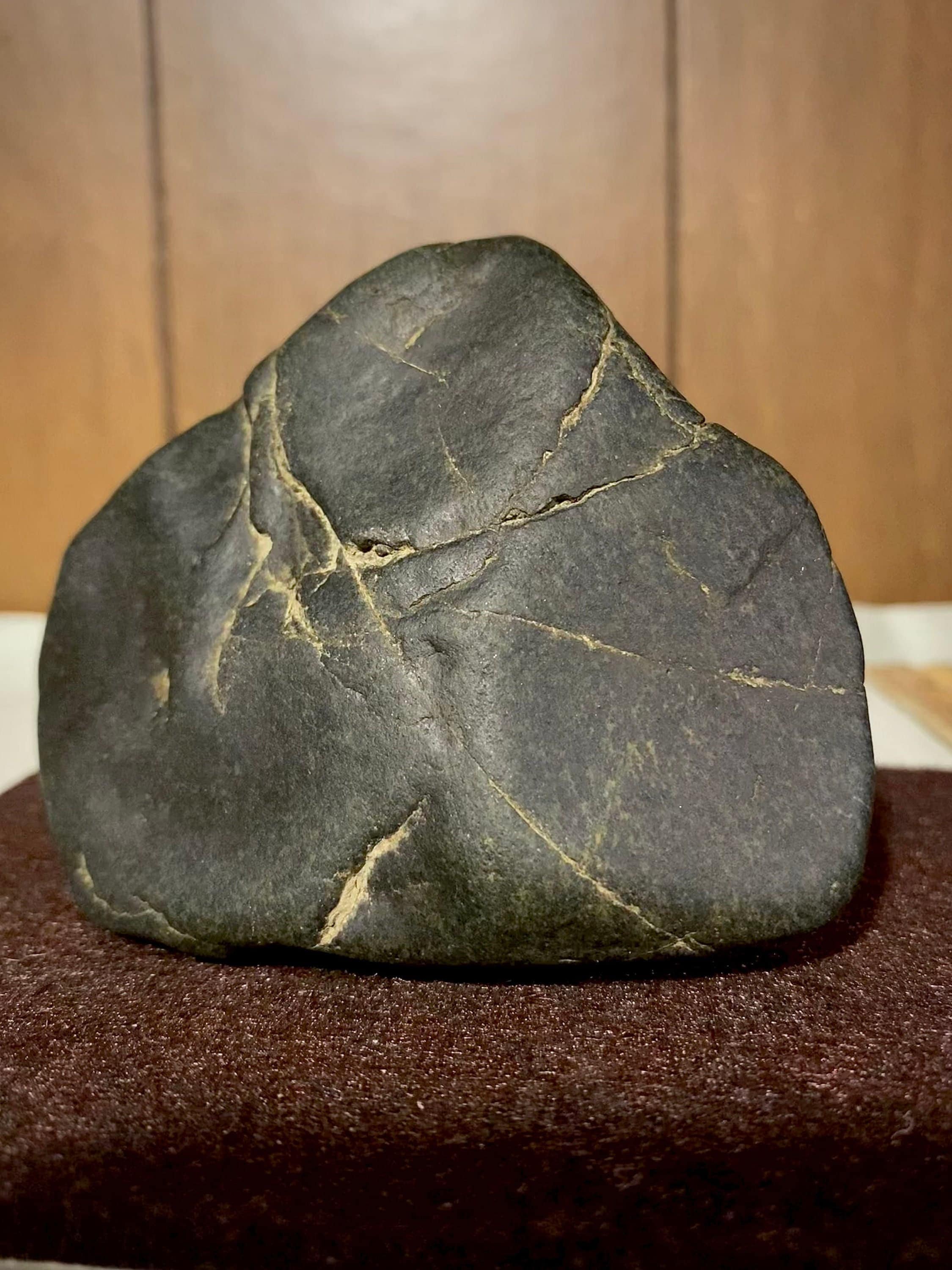In the image, a striking black rock with intricate, golden-yellow veins runs through its numerous cracks is prominently displayed in a museum setting. Positioned on a dark-brown to almost dark-red carpet, the stone exudes an aura of antiquity and significance as it rests carefully on a shelf meant for viewing. The backdrop of the display is a wall with a wood-like surface and a rich brown hue, enhancing the overall aesthetic and drawing attention to the artifact. This rock, with its rich coloration and historical ambiance, appears to be an ancient, valuable stone or artifact, thoughtfully showcased for public admiration and study.